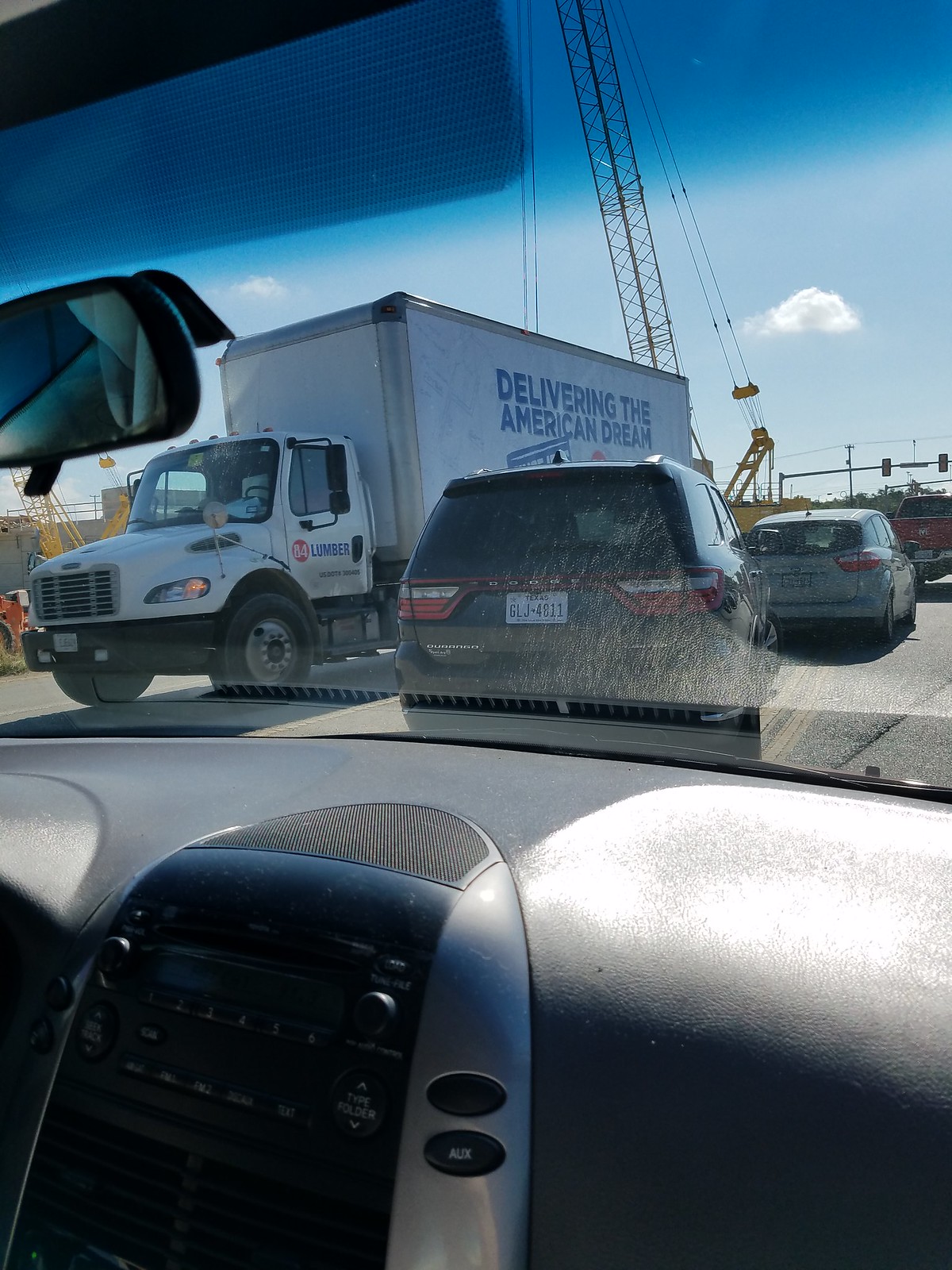Captured from the vantage point of a passenger seat inside a car, this photograph provides a detailed view through the windshield. The interior features are clearly visible, including a dashboard and center console adorned with sleek, light silver metallic accents and an array of buttons. In the lane ahead, several vehicles are lined up, while the opposite lane is dominated by a large white truck bearing the slogan "Delivering the American Dream" in bold blue lettering on its side. The backdrop reveals a picturesque light blue sky speckled with a few small, fluffy white clouds, juxtaposed against the imposing silhouette of a large yellow crane stretching upwards.